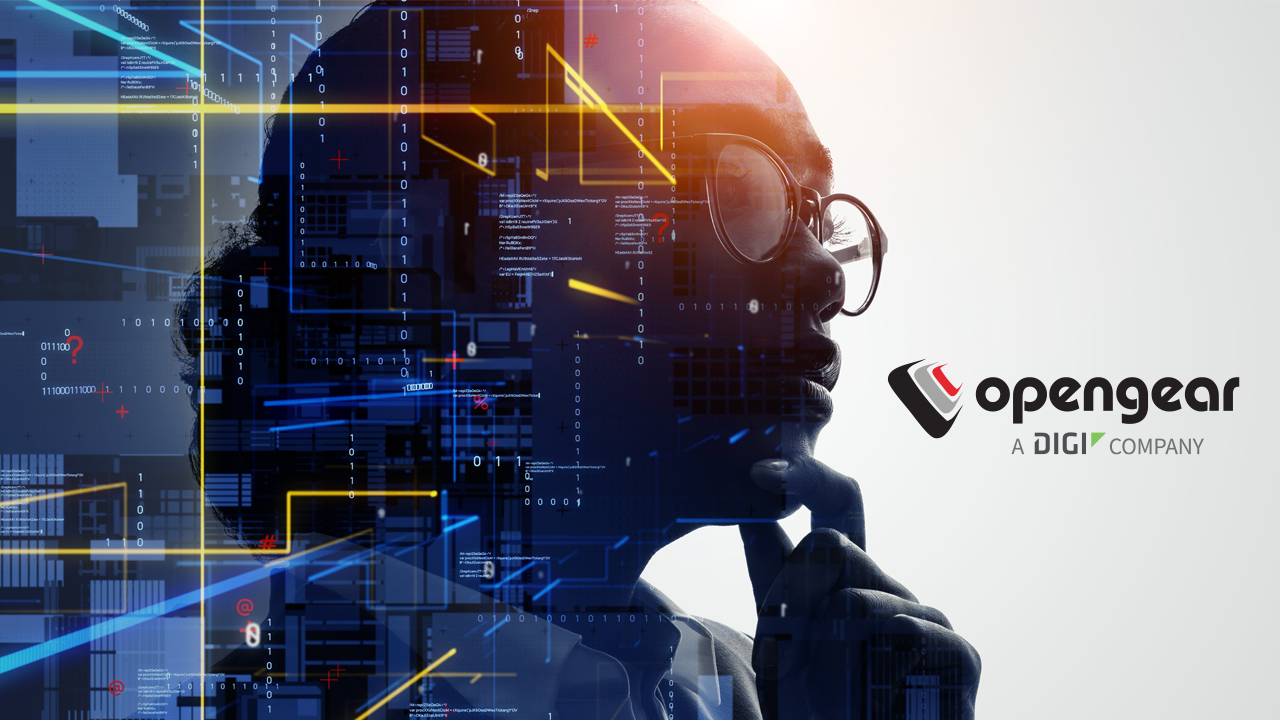The poster features a thoughtful African American woman at the center, wearing glasses and a collared shirt, with her dark hair tied back in a bun. She has her left hand touching her chin, in a pensive pose, gazing into the distance. To her right is the slogan "Open Gear, a digi company," accompanied by a green triangle and a button-like icon. On her left, an abstract depiction of computer networks extends across the background, filled with blue and yellow lines, zeros and ones, question marks, and plus signs, evoking the digital inner workings of software. This combination of human contemplation and digital complexity highlights the innovative essence of the brand.